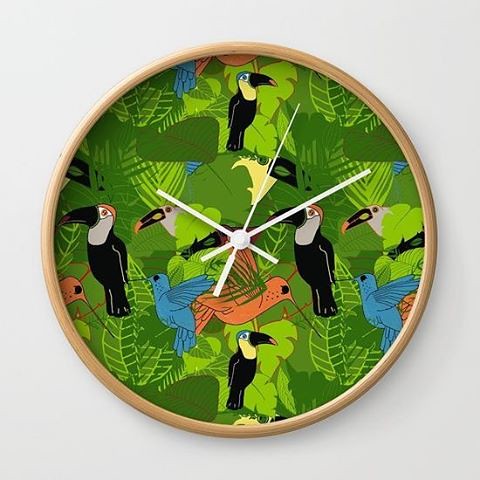This square image features a wooden-framed, colorful clock set against a minimalist off-white background that resembles a wall. The clock's frame, crafted from light brown wood, encloses a vibrant green dial richly adorned with artistic leaf patterns. These leaves vary in shade and texture, showcasing a blend of darker greens with intricate light green veins and smoother green surfaces. Adding to the visual splendor are several ornately depicted birds, each with long beaks and a variety of vivid plumages. These birds come in hues of white, black, black and white, yellow, blue, red, and green, suggesting a mix of tropical species and more familiar birds. The clock’s hands – hour, minute, and second – are elegantly rendered in white, standing out against the colorful and detailed backdrop.